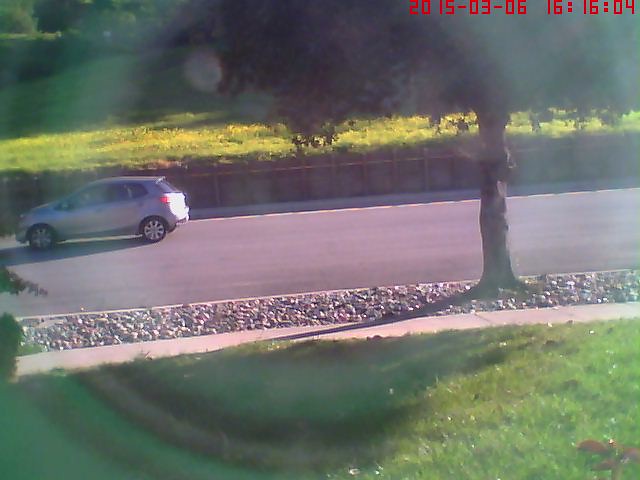The image, captured by a home CCTV camera on March 6, 2015, at 16:16:04, depicts a residential front yard and a section of the street beyond. The foreground features a well-maintained green grass lawn leading to a white concrete sidewalk that runs left to right. Beyond the sidewalk is a gravel and pebble path where a bushy tree is planted, casting shadows over the area. The gray asphalt road, which runs perpendicular to the sidewalk, is bathed in bright sunlight, causing a noticeable lens flare with concentric rings of green and purple on both sides of the image. A small silver car, with its rear bumper highlighted by the sun, is visible on the left side of the frame, driving out of sight. The background reveals a light green or yellow grass verge and a fence line, further indicating the direction of the sunlight from the top right. The timestamp, displayed in red text at the top right corner, adds to the sense of a home surveillance setup.